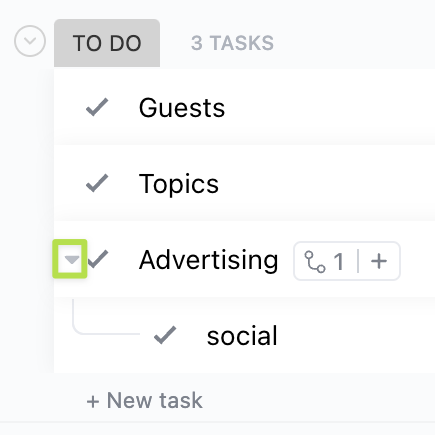The image is a screenshot of a form with a light gray background. In the upper left-hand corner, there's a circle containing a down arrow. Below this, there are two tabs. The first tab, labeled "To Do" in bold, has a gray background. The second tab, labeled "Three Tasks," also has a gray background but with gray text.

The form features three rows. In the first row, there is a gray check mark followed by the word "Guests" in bold. The second row displays a gray check mark next to the word "Topics," also in bold.

The third row is unique. It has a green-highlighted box drawn around a down arrow, indicating that clicking this arrow will expand more information. This box is overlaid on a dark gray check mark. Next to the green-highlighted box, the word "Advertising" is displayed, followed by an ambiguous button that might be a toggle switch. Next to this button, it says "1," with a plus sign button allowing for additional entries.

Directly underneath this, there's a gray check mark next to the word "Social," possibly referring to social media advertising. Finally, at the bottom of the form, there is a plus sign button labeled "New Task," enabling the addition of more tasks.